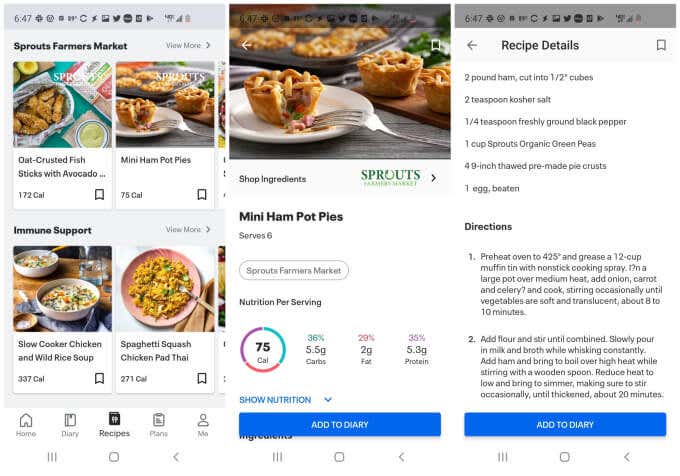**Descriptive Caption:**

This screenshot showcases the results of a search within a mobile app. The left-hand pane is shaded gray and prominently displays "Sprouts Farmers Market" in bold black text. Adjacent to this on the right, there is a "View More" option, accompanied by a small icon.

Below this header, there are two food images, partially obscured but likely depicting deep-fried dishes. The left image is labeled "Oat Crusted Fish Sticks with Avocado," containing 172 calories, complete with an option to bookmark it. The right image denotes "Mini Ham Pot Pies," at 75 calories, adjacent to a Favorites icon.

A banner labeled "Immune Support" stretches across beneath these items, with another "View More" option and the Ford icon in gray to its right. Further down, two more results are presented. The first shows "Slow Cooker Chicken and Wild Rice Soup," containing 337 calories, alongside a Favorites icon. An image of a pink bowl holding food correlates with the label "Spaghetti Squash Chicken Pad Thai," consisting of 271 calories, also accompanied by a Favorites icon.

At the bottom, the app's navigation bar is visible, featuring icons for Home, Diary, Recipes, Plans, and Me. The Recipes tab is highlighted in black, indicating the current active section.